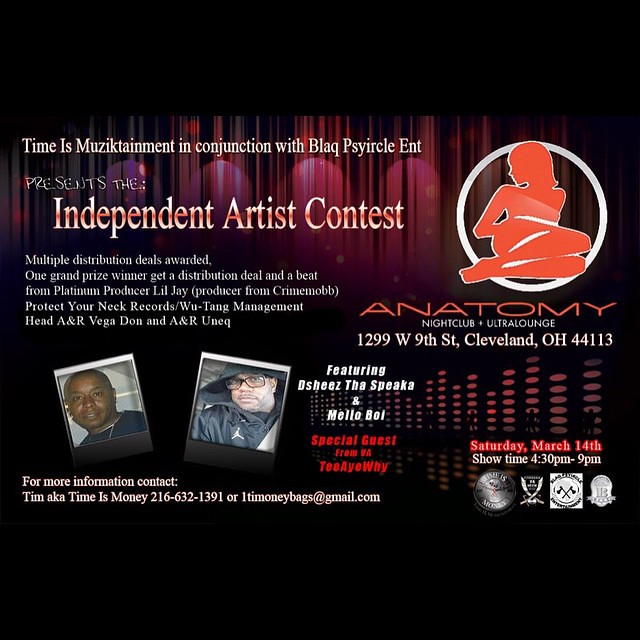This detailed event advertisement poster titled "Time is Musictainment in Conjunction with Black PSY Circle ENT Presents: The Independent Artist Contest" features a combination of bold and informative text. 

At the top left, in striking yellow text, it prominently announces the collaboration, while below in white text, it highlights the event's main attraction: "Multiple Distribution Deals Awarded." The grand prize includes a distribution deal and a beat crafted by the platinum producer Lil' J, famed for his work with Crime Mob. Furthermore, the contest is affiliated with Protect Your Neck Records and Wu-Tang Management, adding a prestigious touch. The head of A&R Vega Dawn and A&R UNEQ will presumably be key figures in the event.

Additionally, the poster visually depicts two men in Polaroid-like images, underscoring its artistic theme. For more information, it directs interested parties to contact Tim, also known as "Time is Money," via phone at 216-632-1391 or email at onetimemoneybags@gmail.com.

On the right side, the silhouette of a woman lying down adds a dynamic visual element, with details of the venue below: Anatomy Nightclub Ultra Lounge, complete with its address. This multifaceted and vividly descriptive poster effectively communicates essential details about the event, promising excitement and opportunities for independent artists.